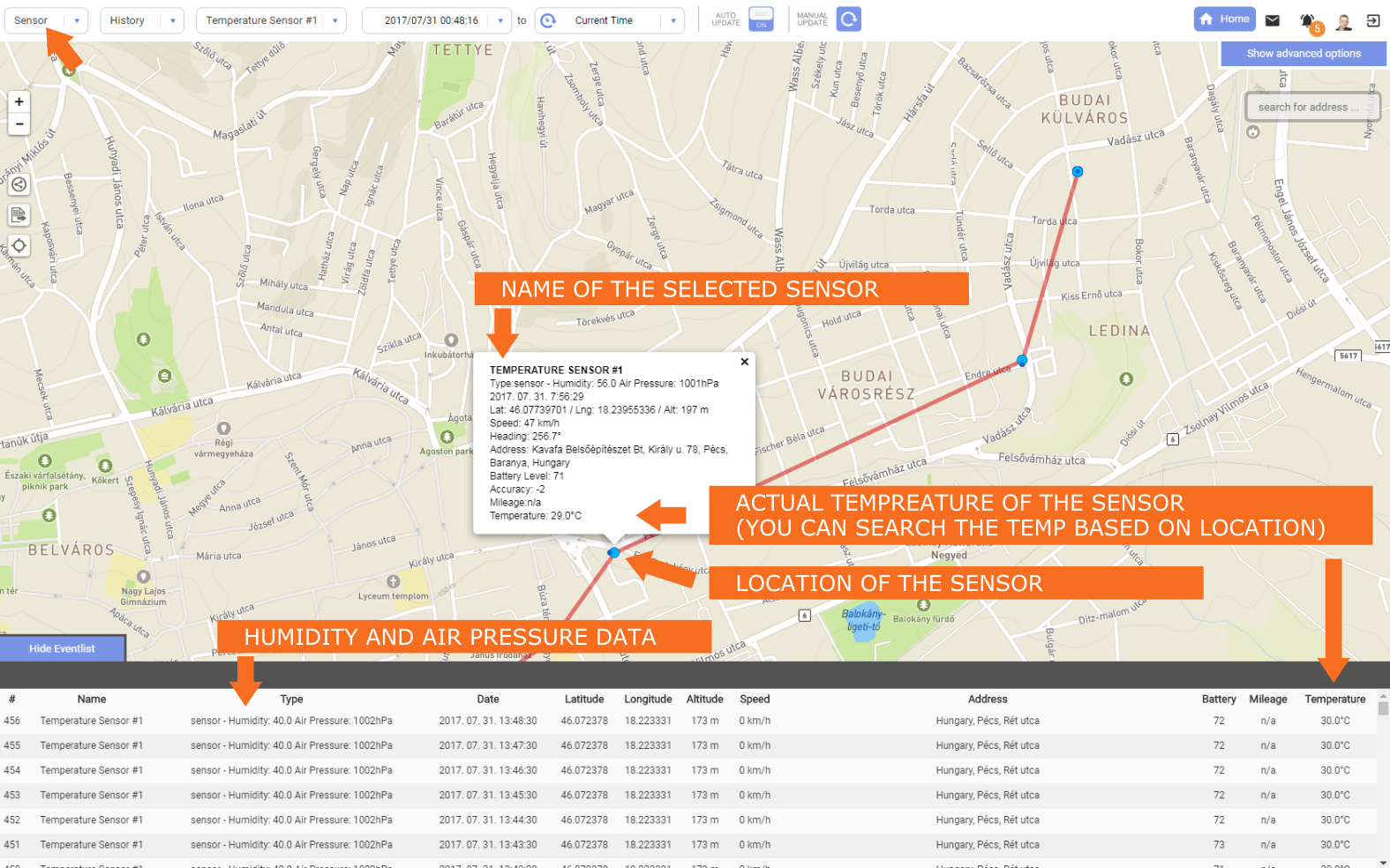The image depicts a detailed sensor monitoring interface. At the top of the page, there is a navigation bar that includes labels such as "Sensor Monitoring," "History," "Temperatures," "Date," "Current Time," along with buttons for "Home," "Email," "Notifications," and "Profile."

The main section of the page features a large, interactive map highlighting the "Name of Selected Sensor." This sensor is identified as a "Temperature Sensor," which is currently registering an actual temperature of 29 degrees Celsius. A blue dot on the map specifies the exact location of this sensor. Additional data provided includes humidity and air pressure readings.

Below the map is a table presenting detailed sensor data:
- Sensor ID: 456
  - Temperature: 29 degrees Celsius
  - Humidity: 40%
  - Air Pressure: 1002 bars
  - Date and Time: January 31, 2017, at 1:48 p.m.
  - Coordinates: Latitude 46, Longitude 18
  - Altitude: 173 meters
  - Speed: 0 (in Hungary)
  - Battery Level: 72%
  - Mileage: N/A
  - Temperature Reading: 30 degrees Celsius

- Sensor ID: 455
  - Temperature: 29 degrees Celsius
  - Humidity: 40%
  - Air Pressure: 1002 bars
  - Date and Time: January 31, 2017, at 1:47 p.m.
  - Coordinates: Latitude 46, Longitude 18
  - Altitude: 173 meters
  - Speed: 0 (in Hungary)

The interface efficiently consolidates a variety of sensor data, offering a comprehensive overview for the monitoring purposes.